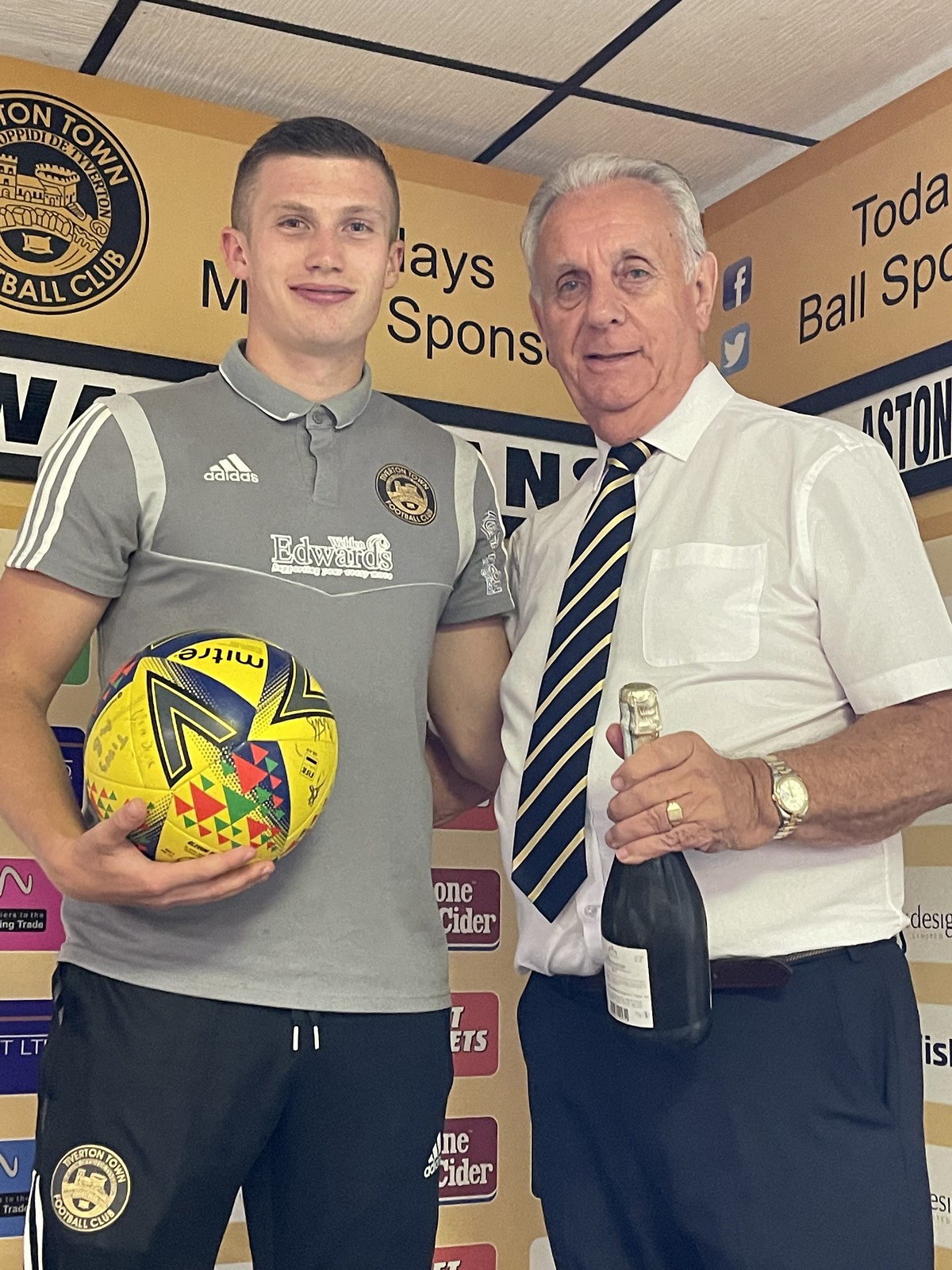This vertically aligned close-up image features two men standing closely together, both with their arms around each other, indicative of a celebratory moment. The man on the left, a young soccer player in his 20s, wears a gray and white collared Adidas polo shirt with "Edwards" written on it, suggesting he is part of a team by that name. He holds a visually striking soccer ball in his right arm, which is predominantly orange and blue, accented with red and green. Dressed in black pants, he exudes a sporty and triumphant demeanor. 

To his right is an older gentleman with short gray hair, smiling warmly down at the camera. He is dressed in a short-sleeved white button-down shirt paired with a striped blue and gold tie, and dark blue slacks. His left wrist is adorned with a gold watch, and he wears a gold wedding band on his left hand, which holds a wine bottle, possibly indicating a celebratory toast. 

The background displays a white tiled ceiling with black borders and walls lavishly decorated in black and gold, featuring various text and logos, possibly sponsors, that add to the festive atmosphere suggestive of a sporting event or victory celebration.